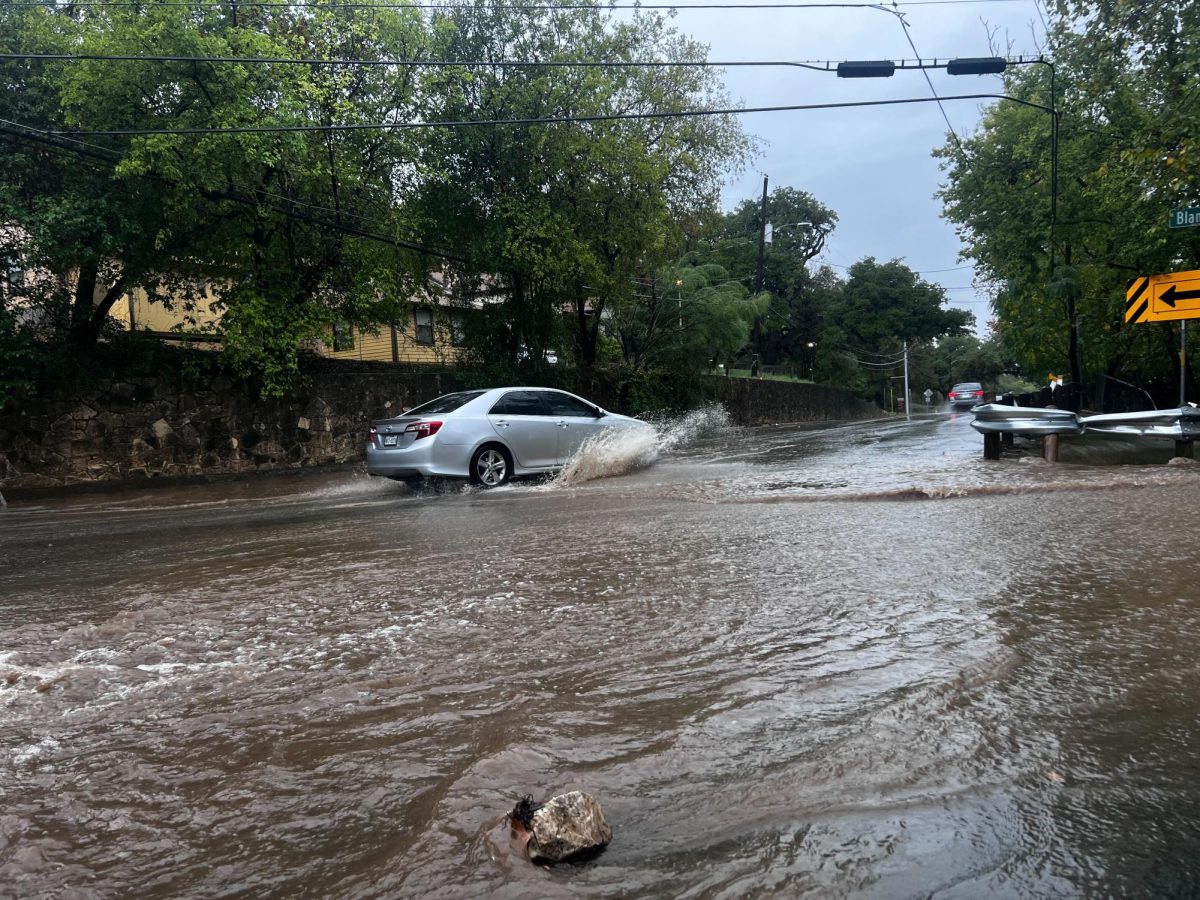The photograph captures a flooded intersection on a black asphalt road with multiple lanes, where parts of the road remain unflooded. Dominating the scene is murky gray-brown water filling the central portion of the intersection, with a large white and gray rock conspicuously located in the dead center at the bottom. A small silver four-door car with silver rims is driving through the floodwaters, which reach partially up its tires and splash out from each side. 

On the right side, the road is bordered by a partially crumpled metal guardrail mounted on small brown posts. Adjacent to the guardrail is a forested area filled with various tall trees and green foliage. A yellow directional sign with a left-pointing black arrow can be seen alongside the guardrail, accompanied by black and yellow stripe markings.

The left side of the image features a six to seven foot tall retaining wall comprised of stones in shades of white, gray, and black. Above this wall are tan houses with black rooftops, nestled amongst green trees and shrubbery. The sidewalk on this side appears wet from the rain. In the background, another darker gray car is visible further up the road, with more trees and signs dotting the landscape.